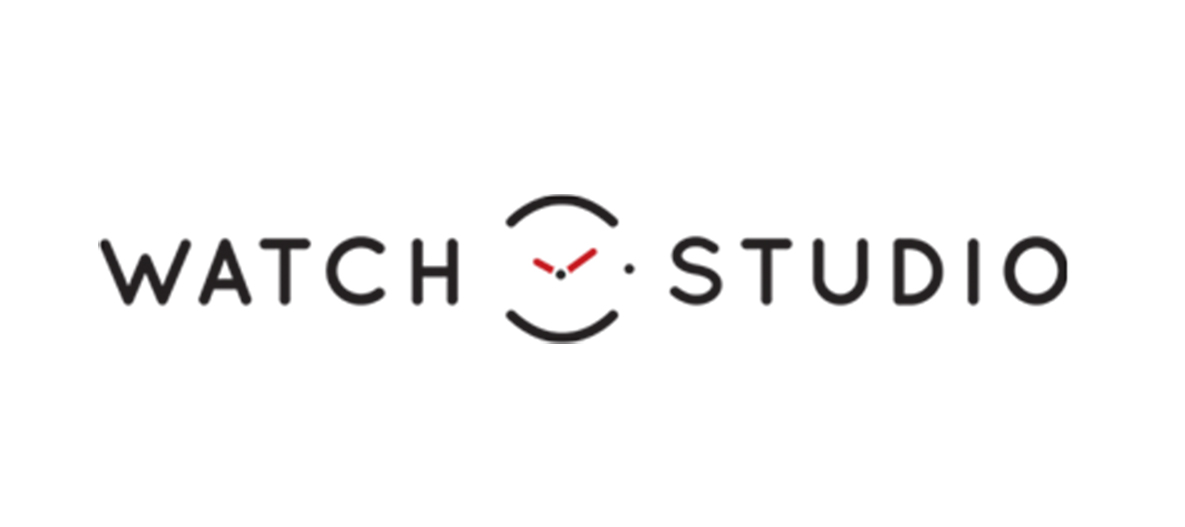The image depicts a simplified business logo set against a plain white background. The logo comprises the words "WATCH STUDIO" in capitalized, curvy, soft-looking text. The text is positioned more towards the top of the image, with "WATCH" on the left and "STUDIO" on the right. Centrally placed between these words is a stylized representation of a watch or clock face. This drawing includes two curved lines; one curving downwards and one upwards, creating a sense of a circular outline. Additionally, there are two red dashes around a central black dot, mimicking the appearance of watch hands – a smaller one and a larger one. The overall design is minimalistic and appears to be a logo for a business.